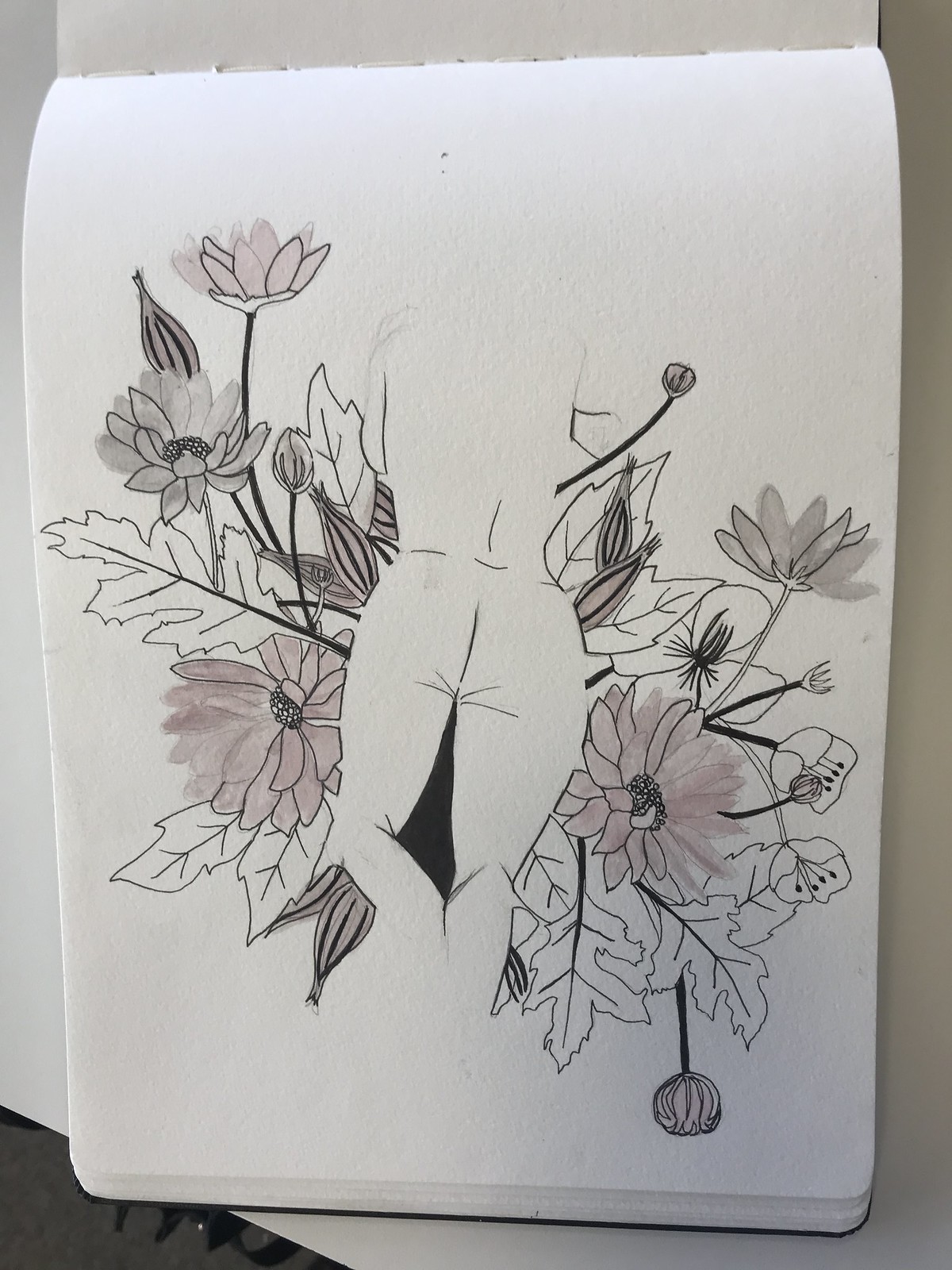The drawing, rendered on a vertical 8 1⁄2 by 11 sketch pad resting on a table, features the incomplete backside of a person. The drawing fades out around the head, shoulders, and feet, leaving the central torso as the focal point. Surrounding the figure, intricately detailed flowers with small petals display subtle hints of pink amidst the predominantly black-and-white composition. The leaves, although resembling those from a maple tree, do not naturally complement the flowers but extend from both sides of the figure, creating an intricate and somewhat surreal visual effect.